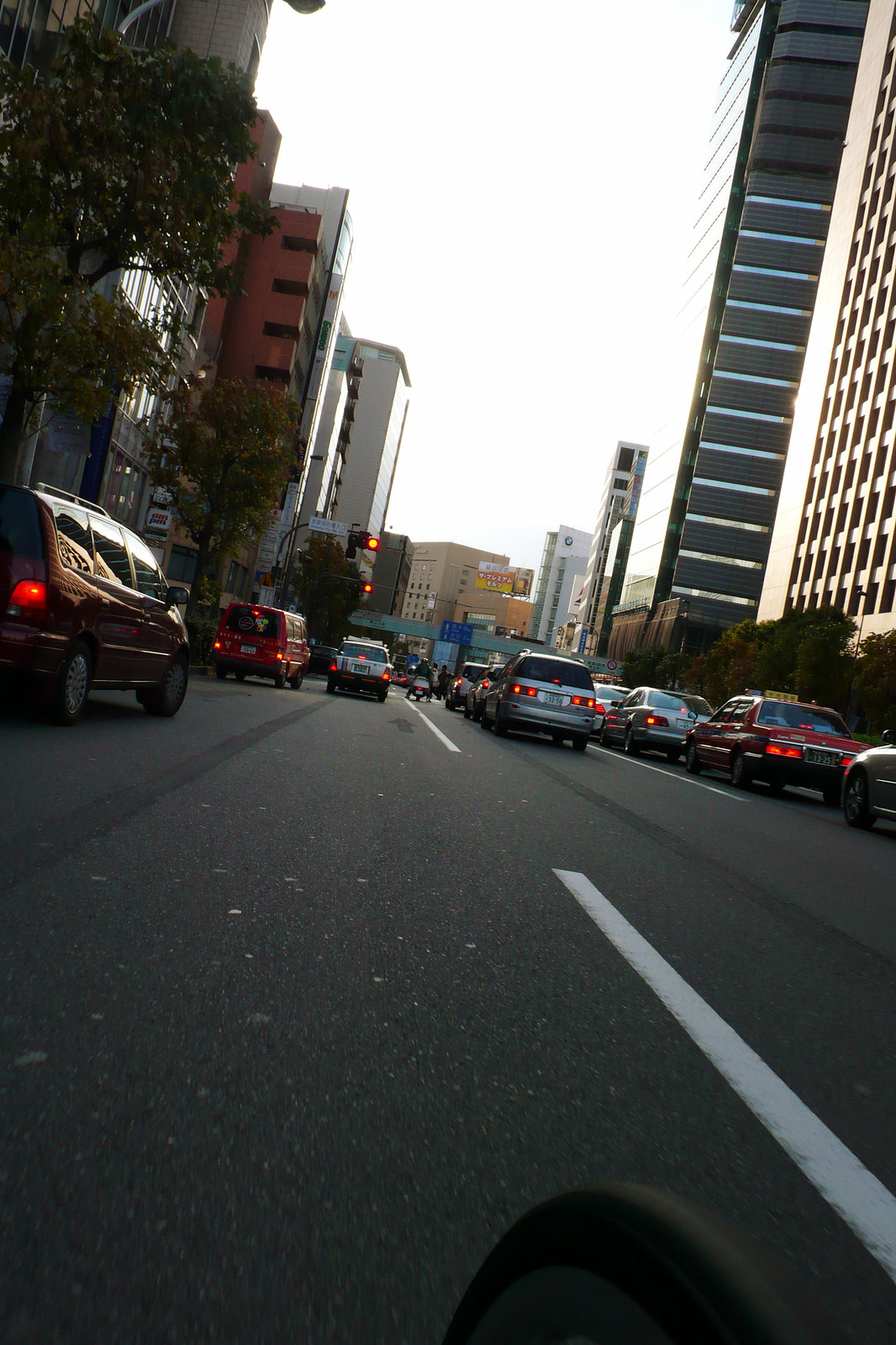The image depicts a typical bustling city street, likely in Japan, captured from what seems to be the perspective of a bicycle or the base of a Segway. The street is congested with a traffic jam, featuring four lanes filled with a diverse array of vehicles. In the leftmost lane, there is a red minivan, followed by a red cargo van, a white Isuzu, a silver minivan, and another white car. Beside them, a bicycle is visible. In the center and right lanes, there are a red taxi, a silver Isuzu, and another white Isuzu. Up ahead, two people are seen crossing the street near the end of the traffic.

The backdrop is dominated by towering skyscrapers on both sides, including a very tall white and silver building on the right-hand side, characterized by numerous windows. On the left, a mix of architectural styles is evident with structures ranging from a reflective glass-fronted building to a more traditional red brick building, a large white building, and more. The overpass in the distance hints at a train route running across it.

The sky overhead is a glaring white, indicating a bright yet cloudy day. Trees are sparsely placed on the left side, adding a hint of greenery to the urban landscape. Distant billboards and more skyscrapers add to the cluttered yet vibrant ambiance of this typical city scene.